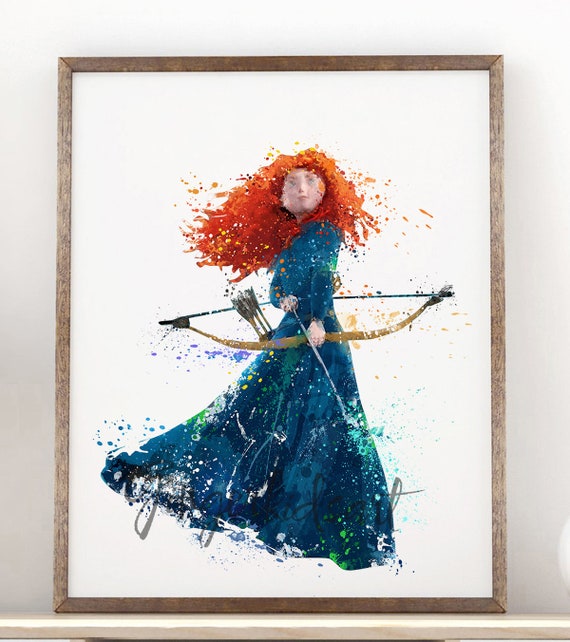In this image, there is a detailed illustration, possibly computer-generated, of Merida from the Disney movie "Brave." She is depicted with her fiery red hair cascading around her face and wears a dark marine blue dress with hints of green and lighter blue accents. Merida is holding a bow at her midsection with one arrow nocked, though the bowstring is not fully drawn, suggesting a moment of poised readiness. Several additional arrows are visible in a quiver attached to her back. This captivating portrait is rendered in an almost splatter paint technique, giving it a dynamic and vivid appearance. The background is stark white, emphasizing Merida's striking figure, and the painting is framed with a simple thin wooden frame. The image appears to be mounted on a white or very light wood shelf against a matching white wall. There is a signature faintly visible at the bottom of her dress, blending subtly with the fabric's texture.